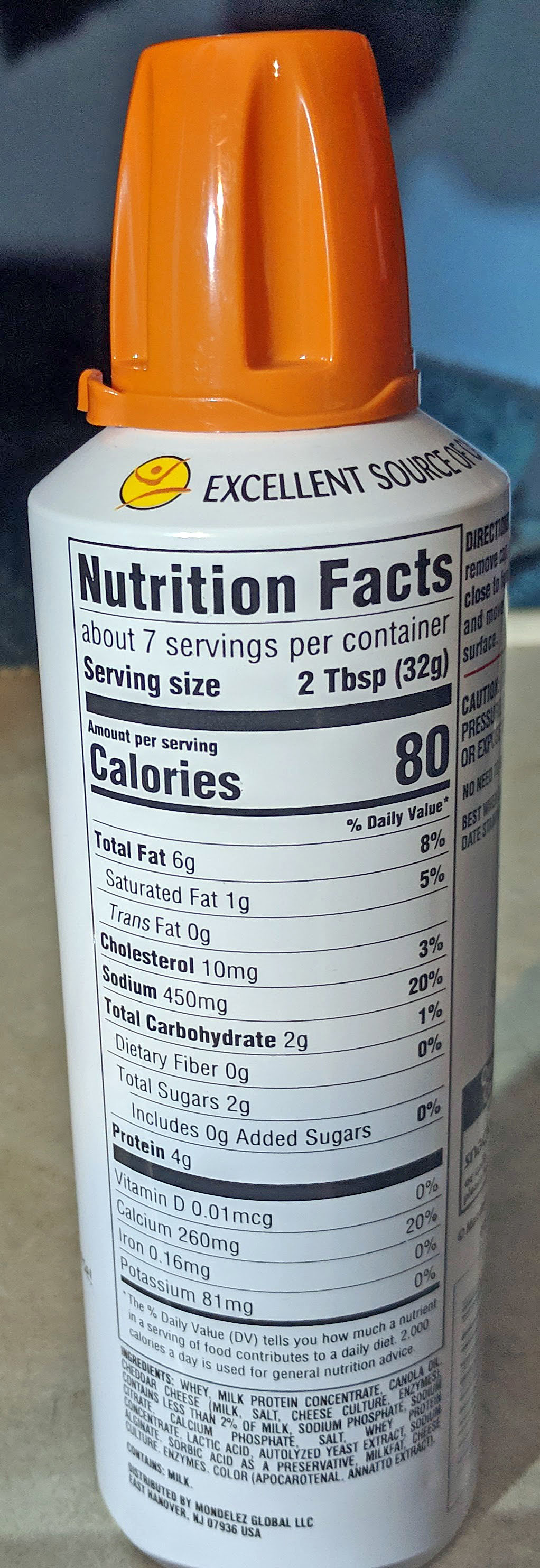The photograph captures a cylindrical food container placed on a flat, gray surface indoors. The background is a blurred blue, making it difficult to distinguish any specific objects or elements. The container is predominantly white with a vibrant orange cap. Its label features black text, including a visible nutrition label. At the top of the label are the words “Excellent Source,” though the remainder of the phrase is obscured as it wraps around the side of the cylinder. Below this, "Nutrition Facts" is prominently displayed, detailing that the container holds about 7 servings, with each serving size being 2 tablespoons (32g) and containing 80 calories. The nutrition label also lists whey milk protein concentrate as the primary ingredient, followed by canola oil and other components.